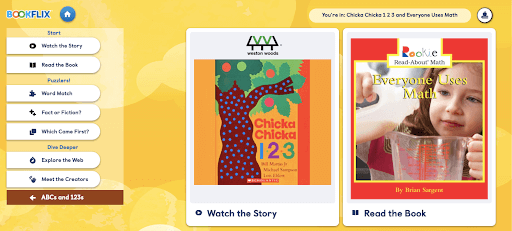The website features a vibrant yellow design and contains several images. One prominent image depicts a young girl holding a measuring cup, and another image showcases the text "Chica Chica, One Two Three, Watch the Story" with a purple animated background. The website appears to cater to young children, offering interactive elements such as books and stories for them to explore and enjoy.